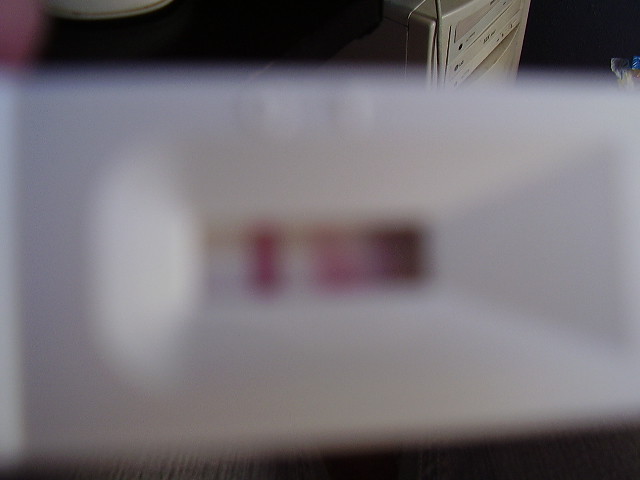This horizontally oriented photograph is extremely blurry, making it difficult to discern specific details clearly. However, it appears to feature a white, rectangular wall mount of some sort, possibly with a three-dimensional structure. The center of this mount seems to be transparent, revealing some pink and white lines. Behind this object, there's a dark background with what looks like a tan-colored object, possibly an old PC. The rest of the background remains predominantly black, contributing to the indistinguishability of the overall scene.